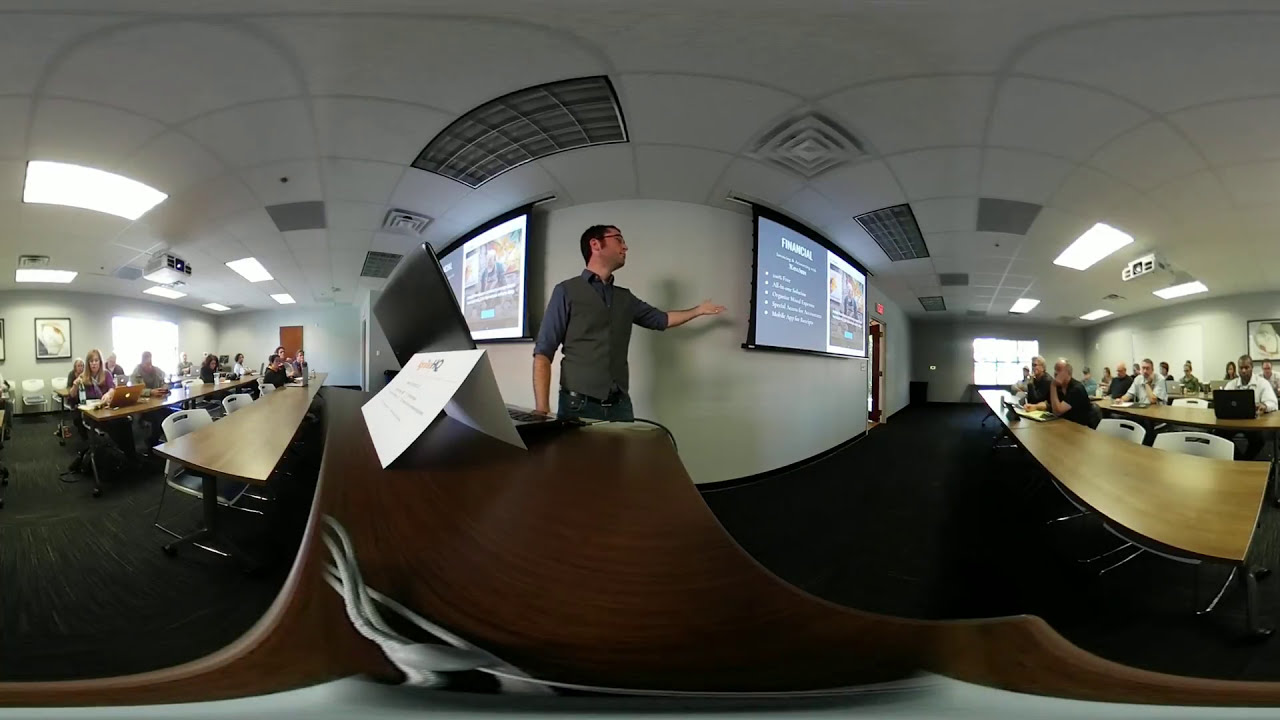In this wide-angle indoor photograph, a group of adults are attentively seated at long wooden conference tables, engaged in a lecture or presentation. The image prominently features a man of Caucasian descent with short black or brown hair, wearing a long-sleeved blue collared shirt rolled up to his elbows, a gray vest, blue jeans, and glasses, standing at the center. He appears to be giving a PowerPoint presentation on financial topics, as indicated by the screen displaying the word "financial" and bullet points. His left arm is extended upwards in a passive gesture, while his right arm rests by his side. On the left, a few attendees, including a woman with brown hair and a water bottle, are seated at tables with laptops. To the right, more participants, including a black individual with a laptop and a white, balding man with a notepad, are similarly focused on the presenter. The setting includes white chairs, brown wooden tables, suspended ceiling with fluorescent lighting, pictures on the walls, and windows flanking both sides of the room, with projectors and a couple of fire exits adding to the detailed backdrop.